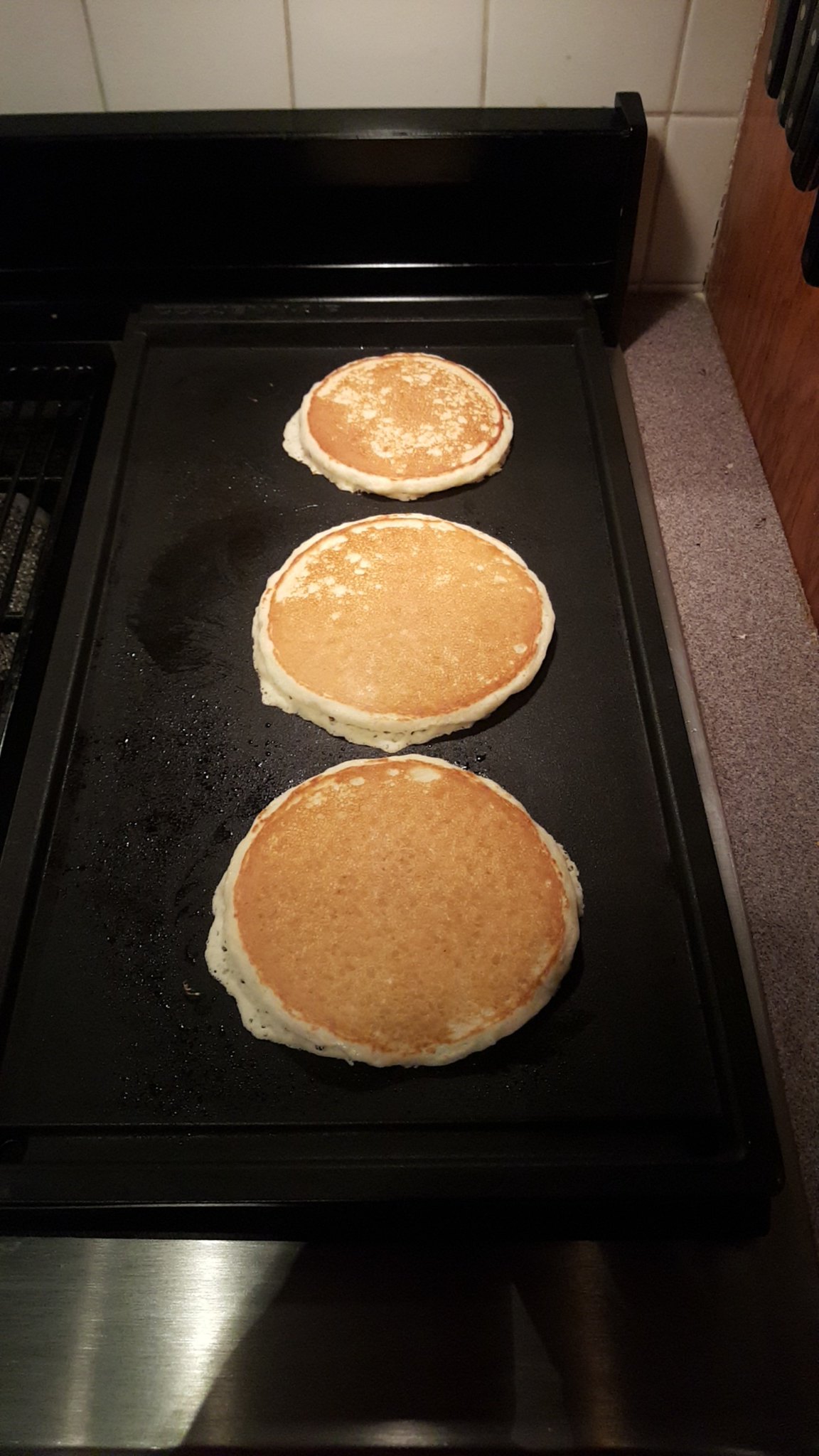In a home kitchen, a top-down photo captures three small pancakes cooking on a large rectangular cast iron griddle that spans two burners on a black stovetop. The pancakes, which have already been flipped, are evenly browned and aligned in a vertical stack on the lightly greased griddle. The stovetop is part of a black stove-oven combo, set against a backsplash of white tiles. To the right, a knife block sits on a countertop, while a wooden cabinet or wall is partially visible in the background. The scene is dimly lit, suggesting a bit of unnatural light, possibly from an overhead vent. The overall composition focuses on the cooking pancakes, exuding a cozy, homey atmosphere.